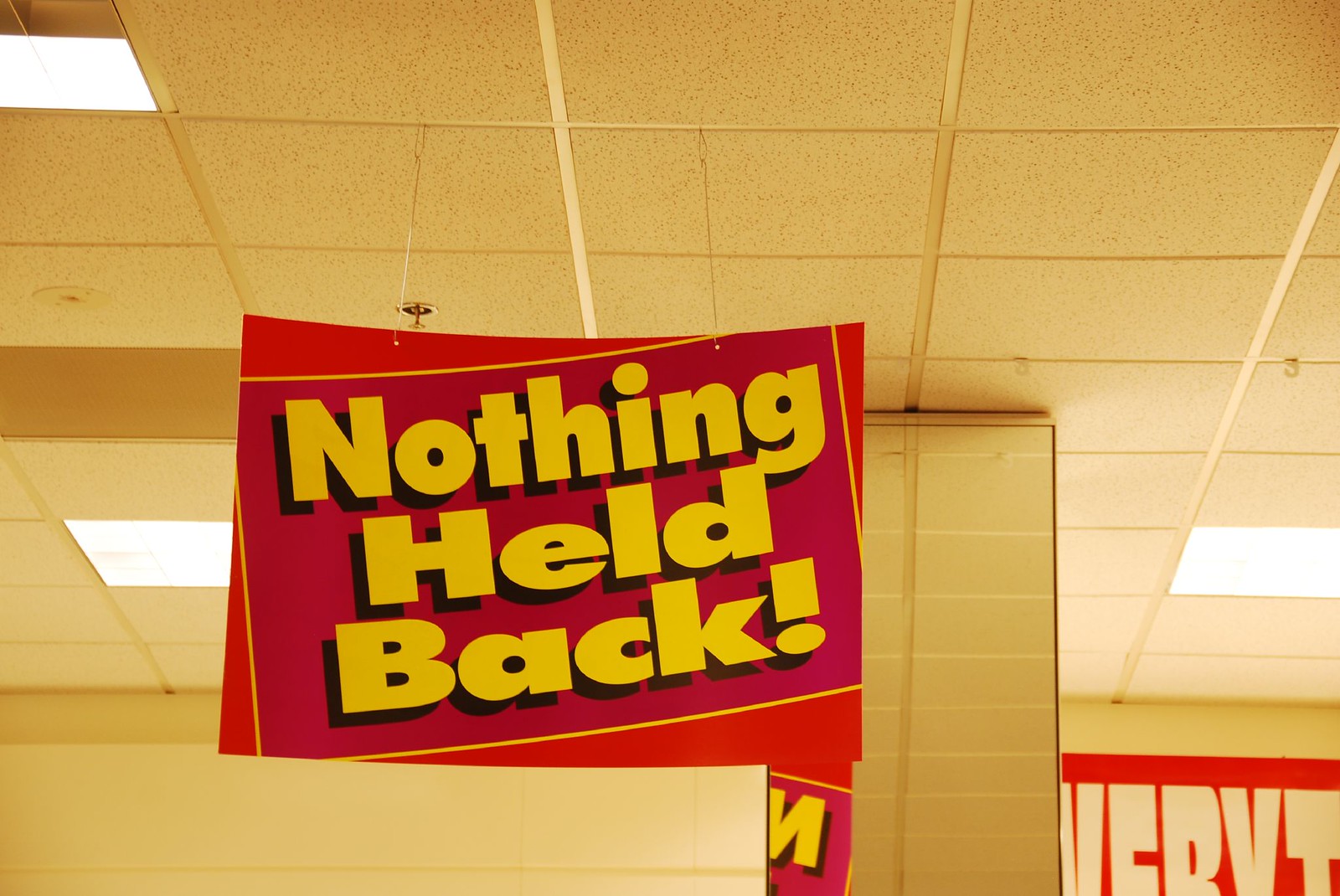The image depicts the interior of a store, viewed upwards towards the ceiling, which consists of tiled panels interspersed with rectangular LED lights. Dominating the scene is a large square sign hanging centrally from wires attached to the ceiling. The sign has a yellow border with a purple interior and features bold yellow lettering that reads "Nothing Held Back!" The walls visible around the sign appear to have a yellowish hue with horizontal paneling. A portion of a red sign with white text is noticeable in the bottom right corner. Overall, the scene is suffused with a warm yellowish tone.